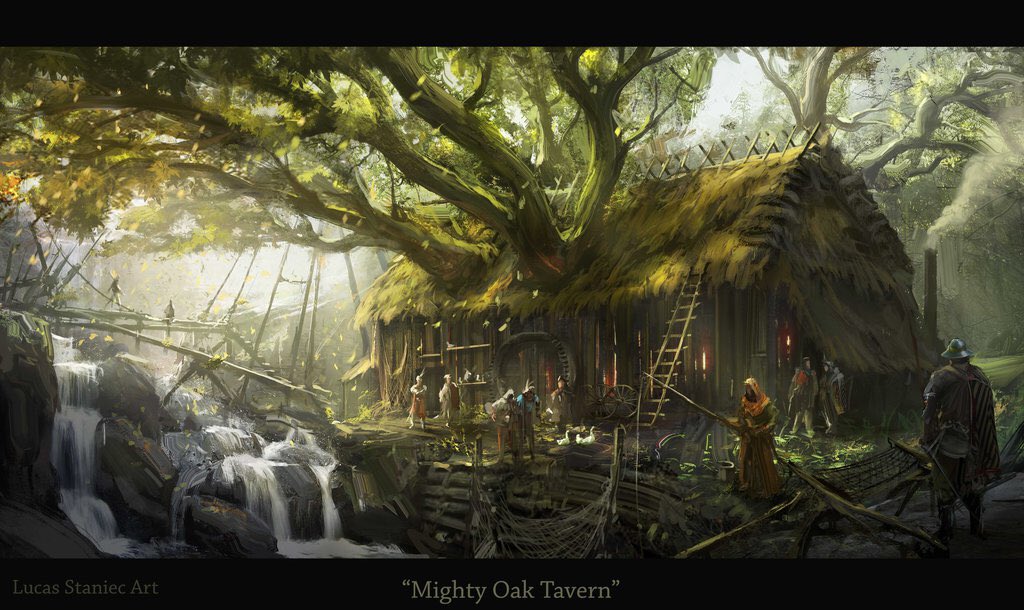This intricate illustration, titled "Mighty Oak Tavern" by Lucas Staniak Art, portrays a rustic tavern scene set in a medieval fantasy world. Framed by black bars at the top and bottom, the image showcases a charming wooden building with vertical dark brown slats and a yellowish-green straw roof, from which colossal oak trees burst through, their branches heavy with smudged yellow-green leaves. To the left, a rocky shallow waterfall tumbles down gray, smudged rocks, with a simple wooden bridge spanning the water, supported by a rope arc.

In the foreground, various figures traverse a stone path. On the right, a man adorned in shining armor and a helmet stands out, while to his left, a robed figure in orange holds a fishing pole, casting into unseen waters below. Surrounding the tavern, which seamlessly integrates the mighty oak into its structure, are more characters dressed in historical attire—helmets, capes, and hoods—evoking an era long past. The ambiance is further enriched by the depiction of some men who appear to be engaged in cutting wood, contributing to the vibrant, bustling atmosphere of this medieval sanctuary.